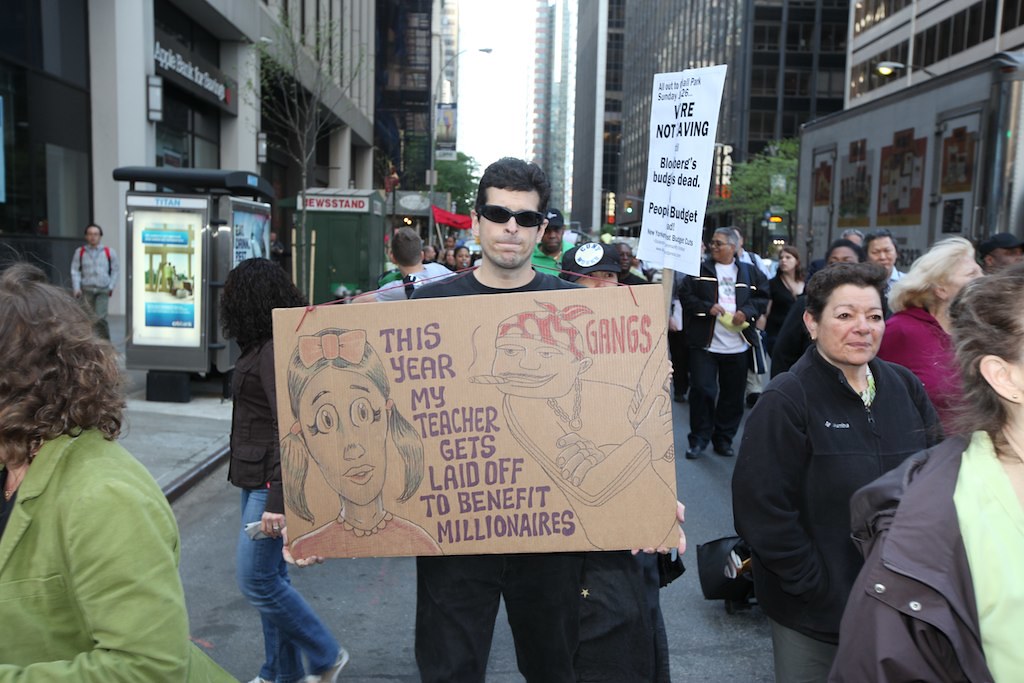The image is a detailed photograph taken on a bustling city street, showcasing a protest scene. Central to the photo is a man in his 30s or 40s, wearing black sunglasses and short black hair, holding a large cardboard sign. The sign contains a hand-drawn sketch on the left of a young girl with black hair in pigtails adorned with a pink bow, and wearing a pink shirt. The middle of the sign reads, "This year my teacher gets laid off to benefit millionaires," in bold purple letters. On the right side, there is a rough sketch of a man smoking a cigar, donning a red and white bandana, a chain around his neck, and three rings on his left hand. Next to this figure, the word "gangs" is written in red. Surrounding the central figure is a crowd of about 15-20 people also holding signs, all marching in the same direction, framed by towering city skyscrapers. The scene vividly captures the essence of a city protest advocating for educational funding.